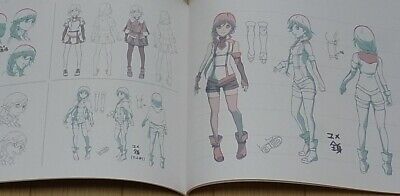The image shows an open art book resting on a tan table, displaying both its left and right pages filled with character sketches. The book's pages, primarily in white, feature detailed drawings and appear slightly blurry. On the left page, there are multiple sketches of what seems to be a female character, likely from an anime, depicted in various poses and expressions—some focusing on the face and others on different outfit designs. The right page showcases a detailed, fully colored character with pink hair, wearing a white shirt, shorts, boots, and fishnet-like sleeves. She is featured in a front view, side view, and back view, primarily drawn in light blue pencil, with accents of dark red and gray. The artwork gives the impression of instructional imagery, possibly a guide on how to sketch anime characters, emphasizing different perspectives and attire details.